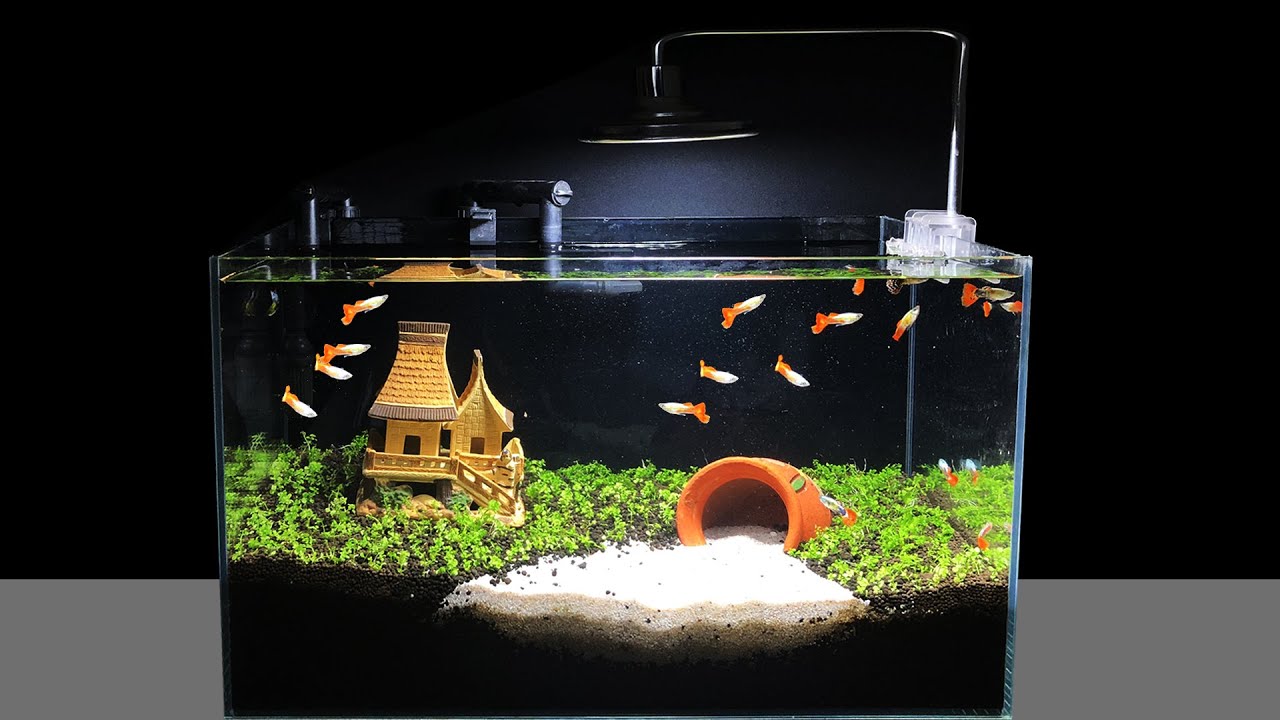This detailed photograph captures a cozy 10-gallon freshwater fish tank situated inside someone's home. The tank, constructed from plexiglass, lacks a lid and features a black background, emphasizing the vibrant colors within. The base of the tank is layered with black sand and pebbles, interspersed with patches of white sand. At the heart of the tank lies a small ceramic vase turned on its side, appearing as if it has spilled its sandy contents. Complementing this are green plants or algae sprouting from the black sand, adding a touch of natural beauty.

A captivating focal point is a small, intricately designed Japanese-style house, enhancing the tank's aesthetic charm. A distinctive feature is the overhanging lamp, attached to a silver metal pole, directing a beam of light right into the center of the tank, ensuring both visibility and a nurturing environment for the fish.

Within this aquatic setup swim approximately 15 to 20 small guppies, identifiable by their white bodies and striking orange tails, suggesting they are all males given their vibrant coloring. Their presence brings lively motion to this meticulously arranged underwater habitat.